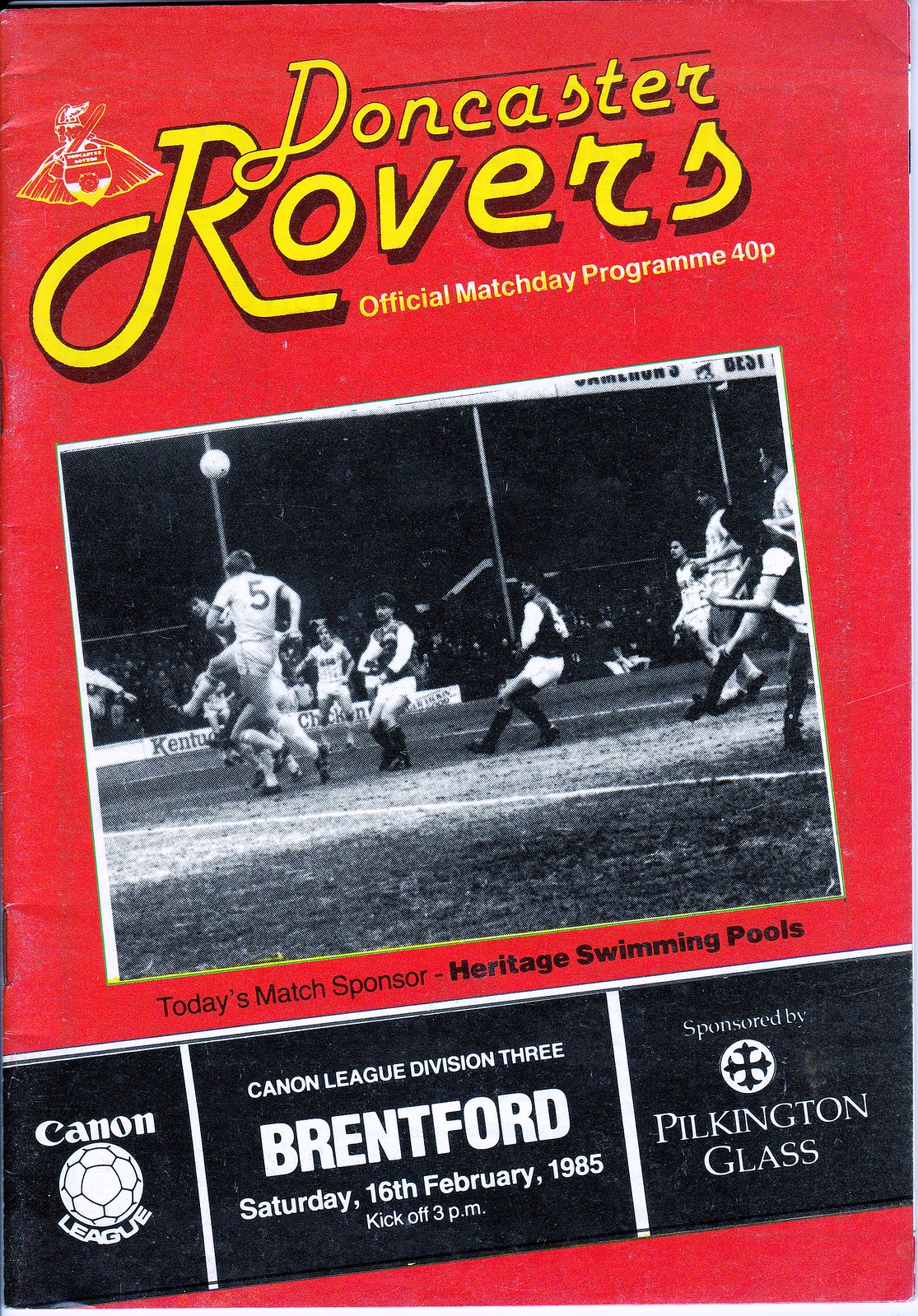The image is the cover of an old Doncaster Rovers official match day program priced at 40 pence. The background is predominantly red with yellow text at the top that reads "Doncaster Rovers" followed by "Official Match Day Program 40P." The top left corner features the team's logo, depicting a Viking with a metal helmet with wings, holding a shield. Centrally, a black and white photograph shows a dramatic soccer moment where a player in a white jersey with the number five is jumping to head the ball while others watch, anticipating its trajectory. Below the photograph, it says "Today's Match Sponsor Heritage Swimming Pools.” The lower section of the cover includes details of the match: "Canon League Division 3," "Brentford," "Saturday, 16th February 1985," and "kickoff 3pm," alongside sponsorship mentions from Pilkington Glass.